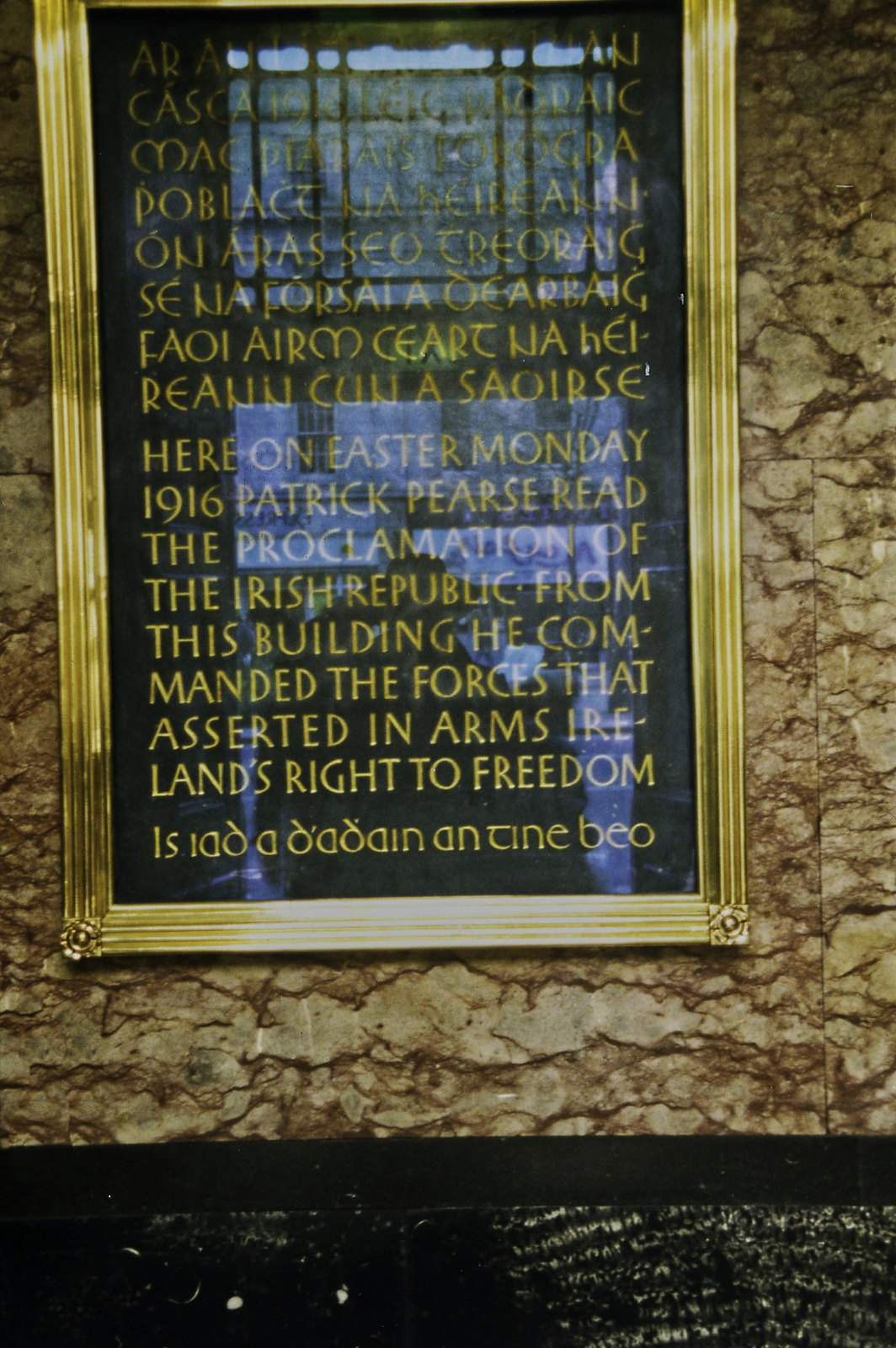This indoor photograph showcases a vertically aligned, framed plaque hanging on a brown, marble or granite wall. The large, gold-rimmed plaque features a background of black with gold text. A noticeable glare, likely from a window or doorway, partially obscures the top portion of the text, which is written in a language other than English, possibly Gaelic. The bottom part, however, is clearly legible and reads: "Here, on Easter Monday, 1916, Patrick Pearse read the proclamation of the Irish Republic from this building. He commanded the forces that asserted in arms Ireland's right to freedom." Below this English text, another line of writing in Gaelic is present. The wall behind the plaque transitions into black tiles at its lower section. The image also captures reflections, including that of the person taking the photograph, highlighting the interplay of light within the space. The primary colors in the photograph are gold, black, and brown.